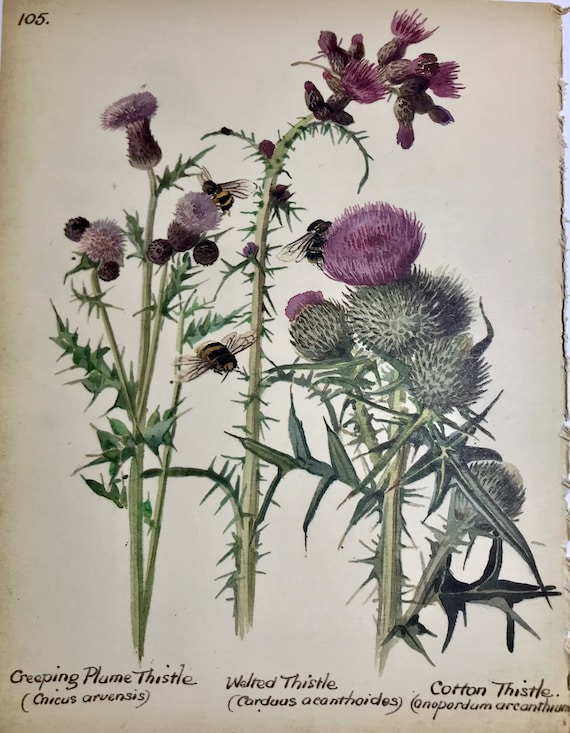This image is a detailed illustration of three different types of thistles: Creeping Plume Thistle (Cirsium arvense), Welted Thistle (Carduus acanthoides), and Cotton Thistle (Onopordum acanthium). All three plants feature spiky green stems and spiky leaves, with round, fluffy purple flowers similar to dandelions but in a vibrant shade of purple. There are also green, spiky-looking buds underneath the flowers. The illustration is highly detailed, depicting bees actively interacting with the flowers, likely collecting pollen. The background resembles a beige cream-colored sketch pad page, adding to the natural and hand-drawn aesthetic of the artwork. Each plant is labeled with both its common and scientific names, although some scientific names are partially obscured or difficult to read, likely due to the handwritten or painted style of the text. The whole scene evokes a botanical study, capturing the intricate beauty and delicate interactions within this thistle community.